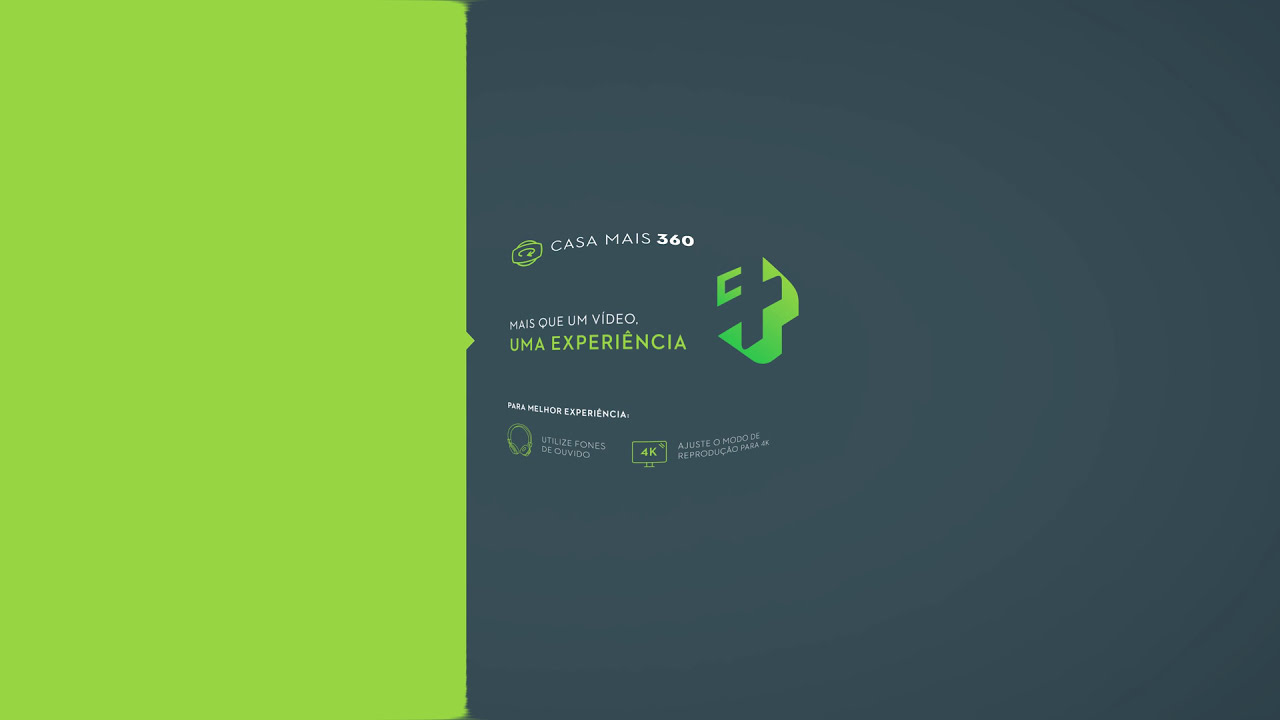The image is a horizontal rectangular poster with a unique presentation, divided sharply between two distinct sections. On the left side, there's a large green rectangle, while the right side is filled with a nearly square, dark blue-green area, approximately twice the size of the green section. In the middle of the image, positioned on the left side of the dark blue-green area, is a section of text not in English. 

At the top of the image, in the green area, there's white text that reads "Casa May 360," accompanied by a logo that blends the green and dark blue-green colors. Below this, in the middle section of the poster, is another piece of text in Spanish: "Make un Video una Experiencia." The bottom portion contains small text that is too fine to be clearly legible. This image likely serves as an advertisement or promotional material combining graphic elements and multilingual text, presenting a striking visual contrast and a call to action.